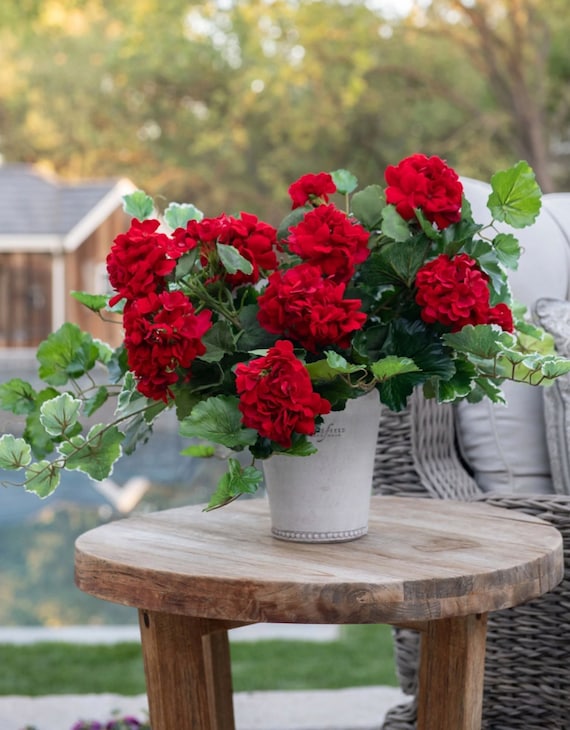The photograph features a charming outdoor scene centered around a rustic white pot filled with a bouquet of vibrant red flowers, likely roses or carnations, nestled among lush green foliage. This pot sits atop a weathered wooden stool, adding to the rustic aesthetic. To the right of the stool is a wicker chair adorned with white cushions, its lattice design contributing to the cozy atmosphere. The background showcases a tree and a quaint house with a brown exterior and blue roof, with indications of a river or pool slightly blurred but discernible. The overall setting exudes a serene, picturesque ambiance, capturing a peaceful outdoor moment.